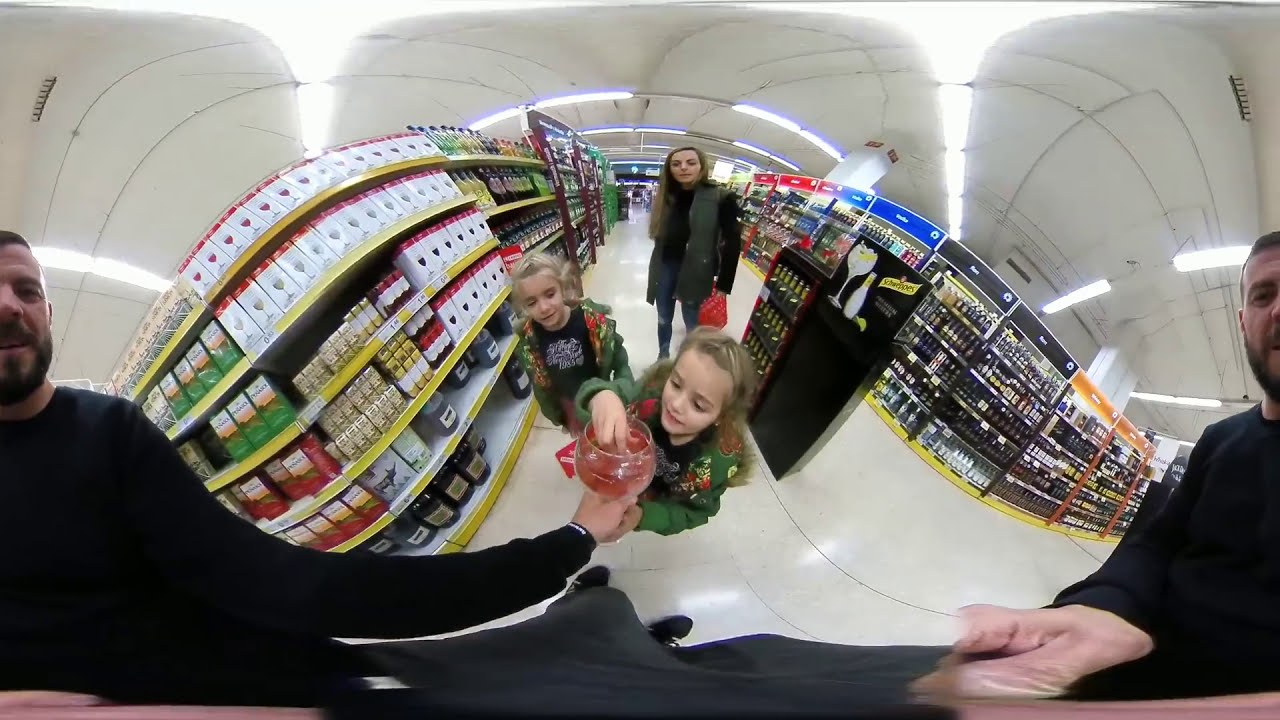This image captures a blurred and distorted indoor scene inside a supermarket, likely taken with a fisheye lens, resulting in a bulging effect towards the center and thinning towards the edges. Dominating the center of the photograph, a woman dressed in black, with long hair, stands on a white tiled floor. Surrounding her on both sides are store shelves laden with various groceries in different colors. In front of the woman, two young girls with long blonde hair, wearing green matching jackets and black shirts with white lettering, are reaching into a large clear wine glass. One of the girls is pulling out a red object, presumably a piece of candy. Interestingly, the man holding the clear wine glass, dressed in a long black shirt with a mustache, beard, and short brown hair, appears twice in the image—his mirrored reflection featuring on both the left and right sides of the photograph. Fluorescent lighting illuminates the white ceiling above, completing the brightly lit store setting.